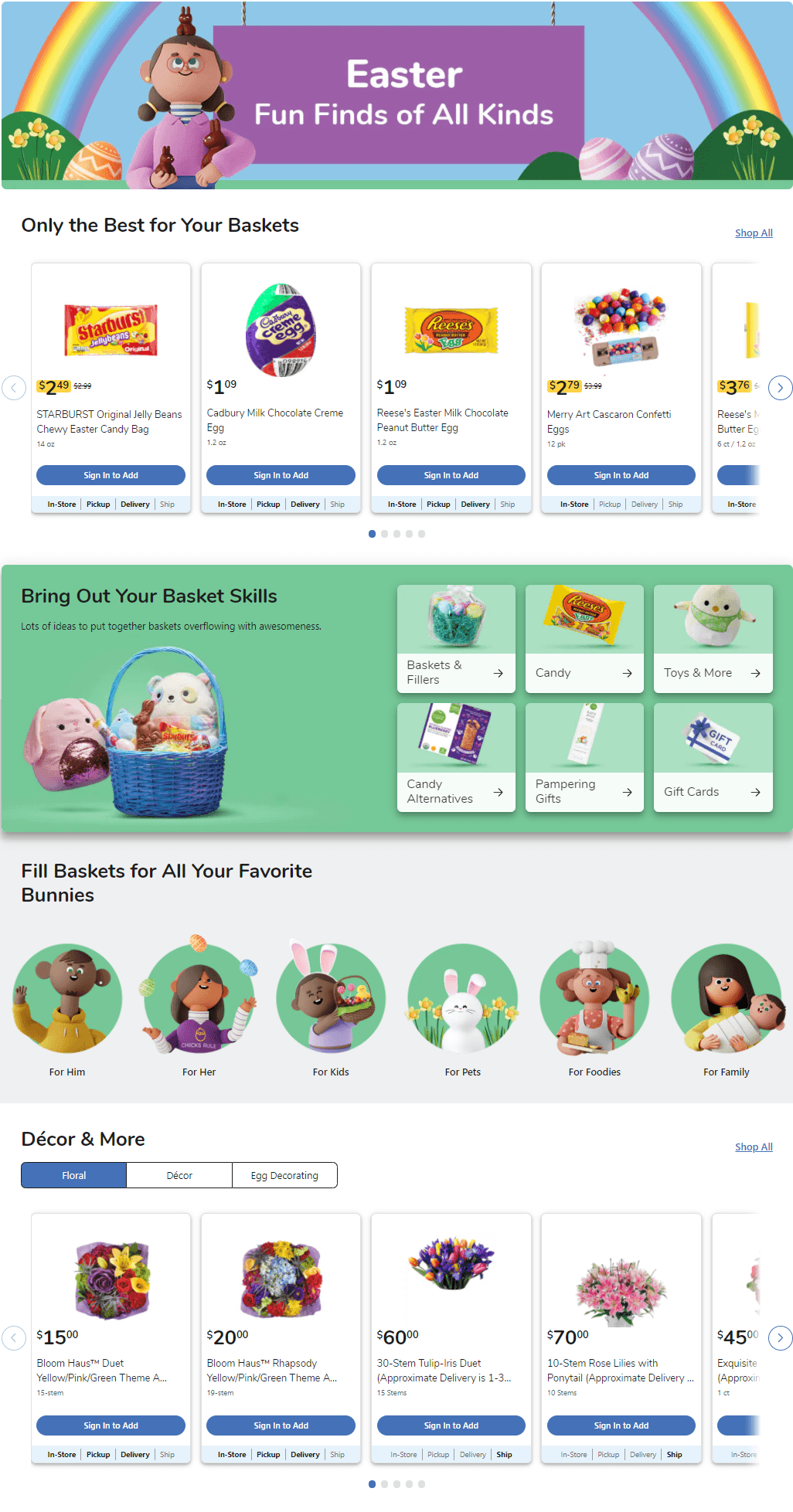Screenshot caption: "A promotional image for Easter-themed products perfect for your holiday baskets. Featured items include Starburst candies, Reese's Peanut Butter Eggs, and colorful candy eggs, priced at $2.49, $9, and $2.79 respectively. Sign in to add these treats to your cart. Enhance your basket-building skills with a variety of items, like a blue basket adorned with pink bunnies. The backdrop is predominantly white with some green accents and floral arrangements at the bottom. Other products are priced variably at $15, $20, $45, $60, and $70. The image also depicts three individuals of African descent, highlighting diversity. Bring out your creativity and fill your Easter baskets with only the best finds!"